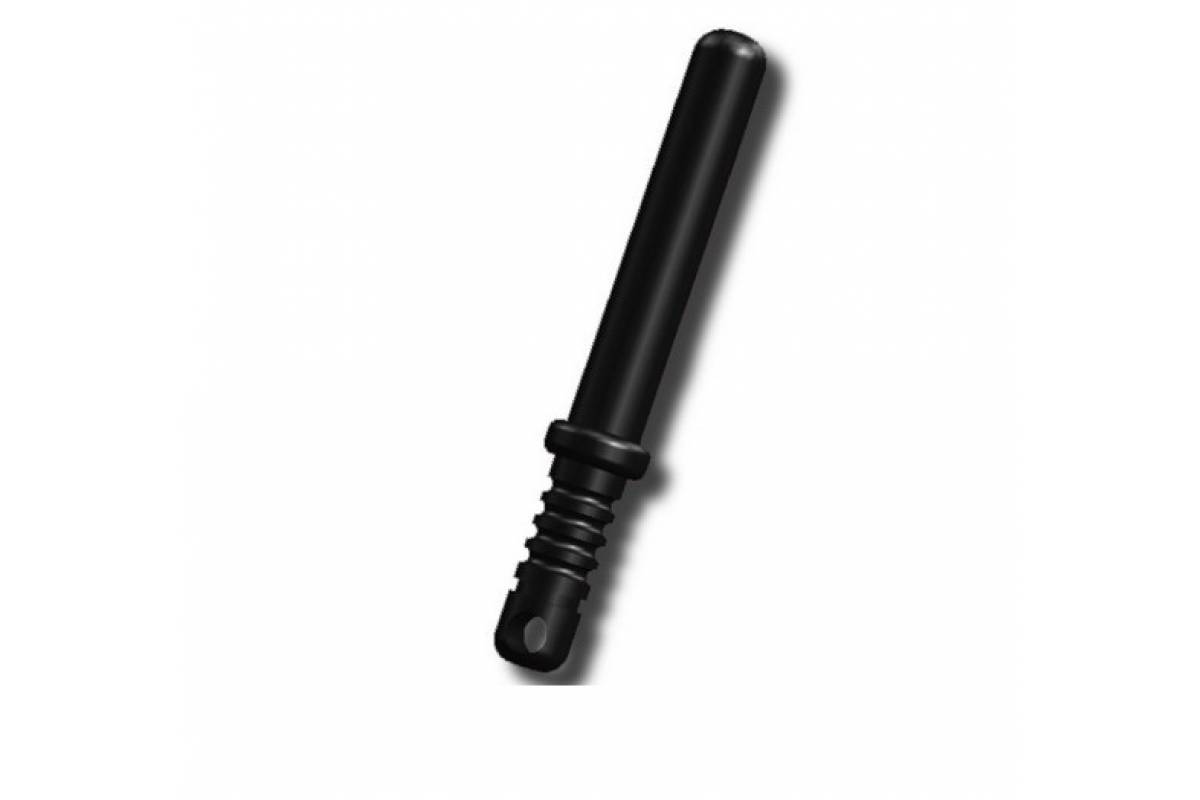The image features a sleek, black police baton set against a white background with no borders or text. The baton is primarily constructed from shiny black plastic, giving it a glossy appearance. Its design mimics that of a short bat or nightstick. The baton includes a handle at the bottom, which has a distinctive grip facilitated by three prominent ribs or ridges encircling it. At the very end of the handle, there's a small, lighter black oval. Above the grip area, a wider piece of plastic protrudes, adding to its sturdy construction. The baton extends into a long, smooth, cylindrical shape, terminating in a rounded top. A shadow cast to the right of the baton emphasizes its texture and the ridges along the grip.